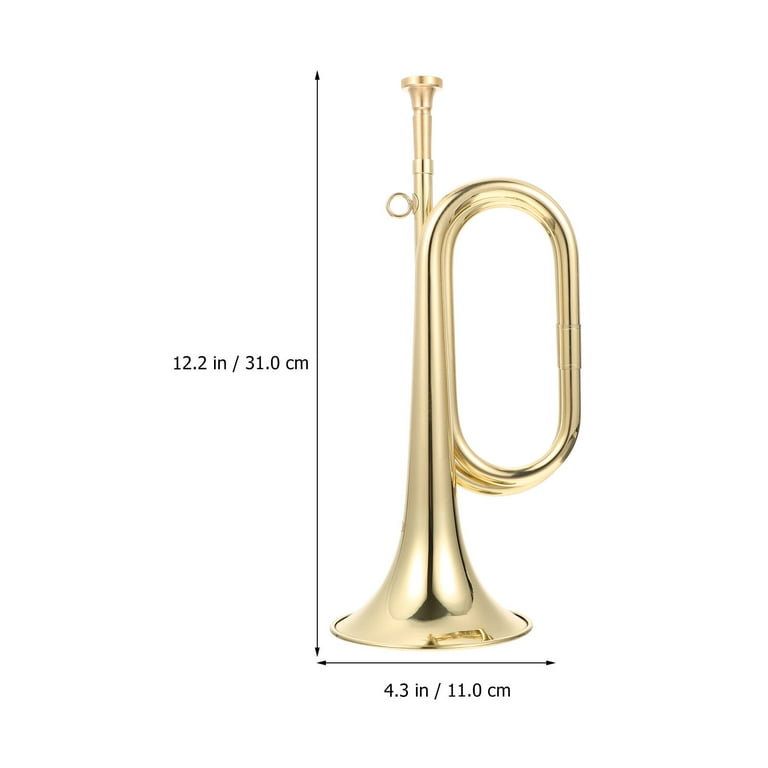This is an image of a shiny golden French horn, crafted from brass, displayed as a typical product shot. The instrument stands upright on its flared bell, from which sound emanates, with the mouthpiece elevated off the white surface, blending seamlessly with the white backdrop. The French horn is meticulously measured, standing 12.2 inches (31.0 centimeters) tall and 4.3 inches (11.0 centimeters) wide. Notably, the gleaming finish of the horn reflects light strikingly. Though keys are not visible from this angle, they may be present on the reverse side of the instrument.